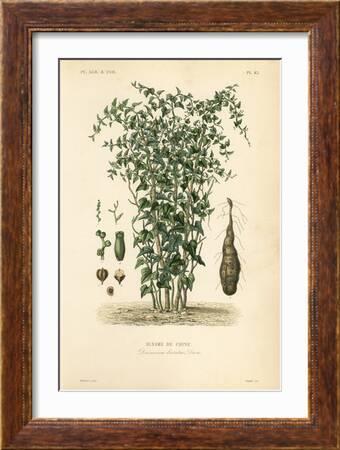This framed illustration showcases a botanical drawing in a brown wooden frame with a white mat. The picture, set against a beige background, features a detailed sketch of a green plant with various components depicted around it. The central plant appears bushy with green leaves and stalks, its top bending slightly. On the right, an illustrated root system, including a tuber with extending roots, is visible, although the ground is represented by a drawing rather than an actual image. The left side displays what looks like seed pods or flowers, laid out in an open space. There is small, illegible text beneath the illustrated soil. The meticulous color work and the detailed presentation suggest a classic botanical art style.